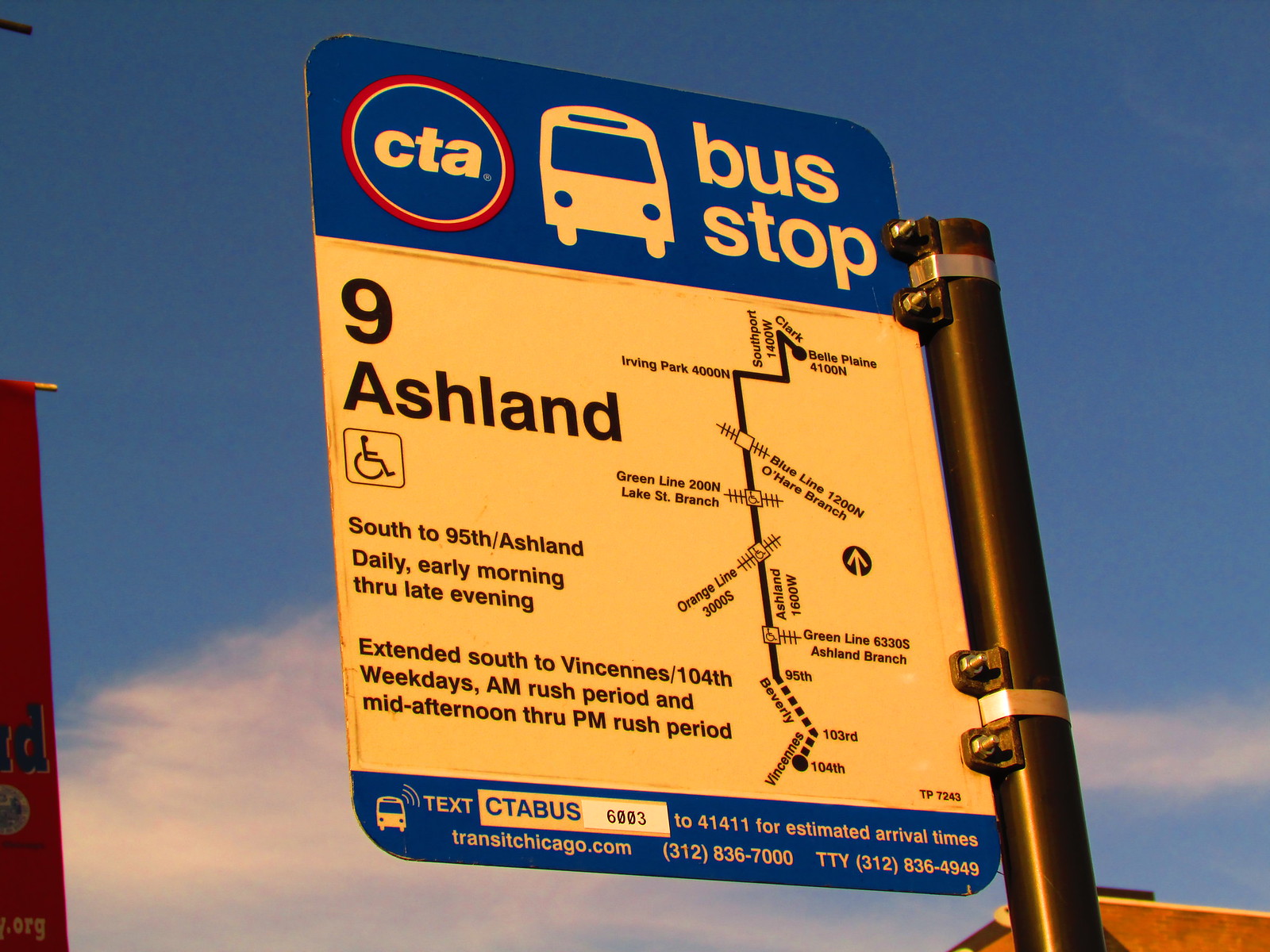The image features a detailed close-up of a bus stop sign against a vibrant blue sky adorned with puffy white clouds. The sign is mounted on a black, round pole. The top portion of the sign consists of a blue banner highlighting a white CTA logo inside a red circle and an image depicting the front of a bus in white. Below this, the sign reads "Bus Stop" in white lettering with a large number "9 Ashland" and a wheelchair symbol indicating accessibility. To the right of these details is a map displaying the bus route. Further information on the sign describes the bus service: it travels south to 95th/Ashland daily from early morning through late evening, with extended services to Vincennes and 104th on weekdays during AM and PM rush periods. Additional text at the bottom of the sign provides a contact number for estimated arrival times (text CTA bus 6003 to 41411) and lists the Transit Chicago website (transitchicago.com) as well as phone numbers (312-836-7000 and TTY 312-836-4949) for further inquiries.